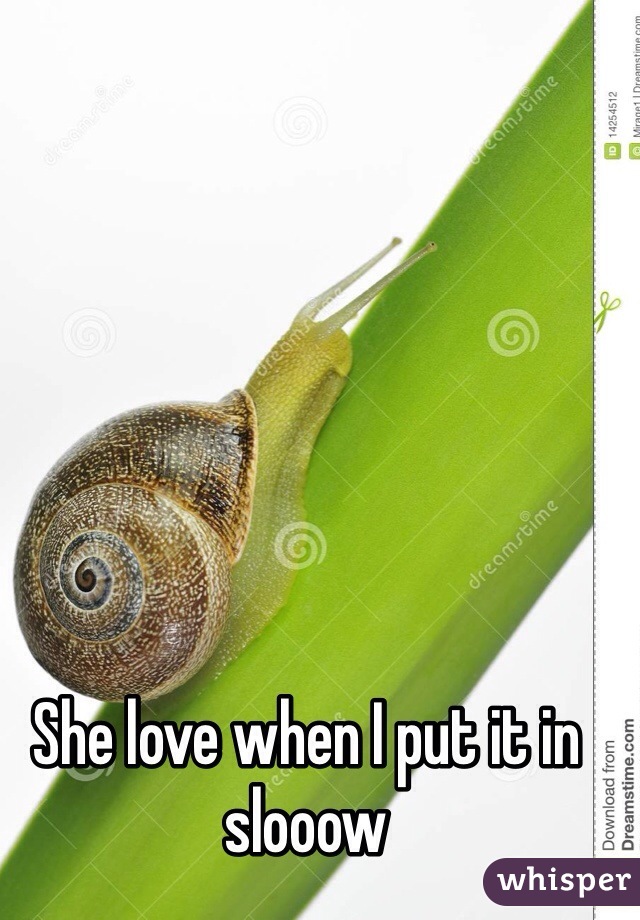The image showcases a large snail with a speckled brown and tan shell and light green body, prominently crawling up a bright green, diagonal stalk against a white background. The snail, central to the image composition, has two antennas extending from its head. Below the snail, in a playful meme-like style, white text with a black outline humorously reads, "She love when I put it in slooow," referencing the snail's slow movement. The image is watermarked with "Dreamstime" and their swirly logo, indicating it is a stock photo from Dreamstime.com. Additionally, the bottom right corner features a purple symbol bubble labeled "Whisper," with the text "download from Dreamstime.com" written vertically. An ID number, 1-425-4512, is situated in the image's upper right corner.